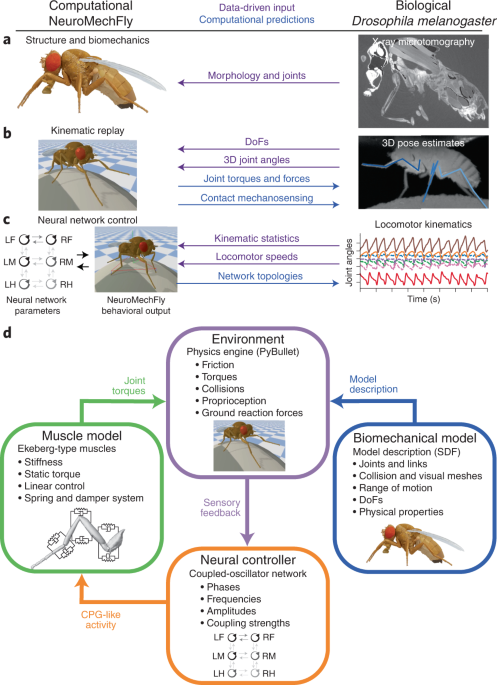The scientific diagram provides a comprehensive depiction of the life cycle and ecological impact of a particular species of fly, specifically the biological *Drosophila melanogaster*, often used in computational and biomechanical studies under the term "Computational Neuro-Mech Fly." The diagram is segmented into several rows labeled A through C, each detailing different aspects of the insect's structure and behavior.

At the top, the heading "Computational Neuro-Mech Fly" is prominent, followed by annotations like "Data-Driven Input Computational Predictions." The first row (A) is dedicated to the fly's structure and biomechanics, highlighting its morphology, joints, and biomechanics, along with detailed x-ray micro-tomography images showcasing the insect's internal composition and 3D pose estimates.

The second row (B) focuses on 'Kinematic Replay,' which involves illustrations of the fly in motion and information on 3D joint angles, joint torques, forces, and contact mechanosensing. These illustrations elucidate how the insect moves and reacts to physical stimuli.

Row C dives into more advanced kinematic statistics, describing locomotor speeds and network topologies. This row also contains images and diagrams that showcase biomechanical modeling, neurocontroller systems, and muscle models that explain the insect's response to various environmental stimuli.

Overall, the diagram integrates various elements like detailed illustrations, x-ray images, 3D pose estimations, and complex biomechanical models to present an exhaustive analysis of the fly’s anatomy, motion, and ecological interactions, highlighting the sophisticated computational methods used in studying this organism.